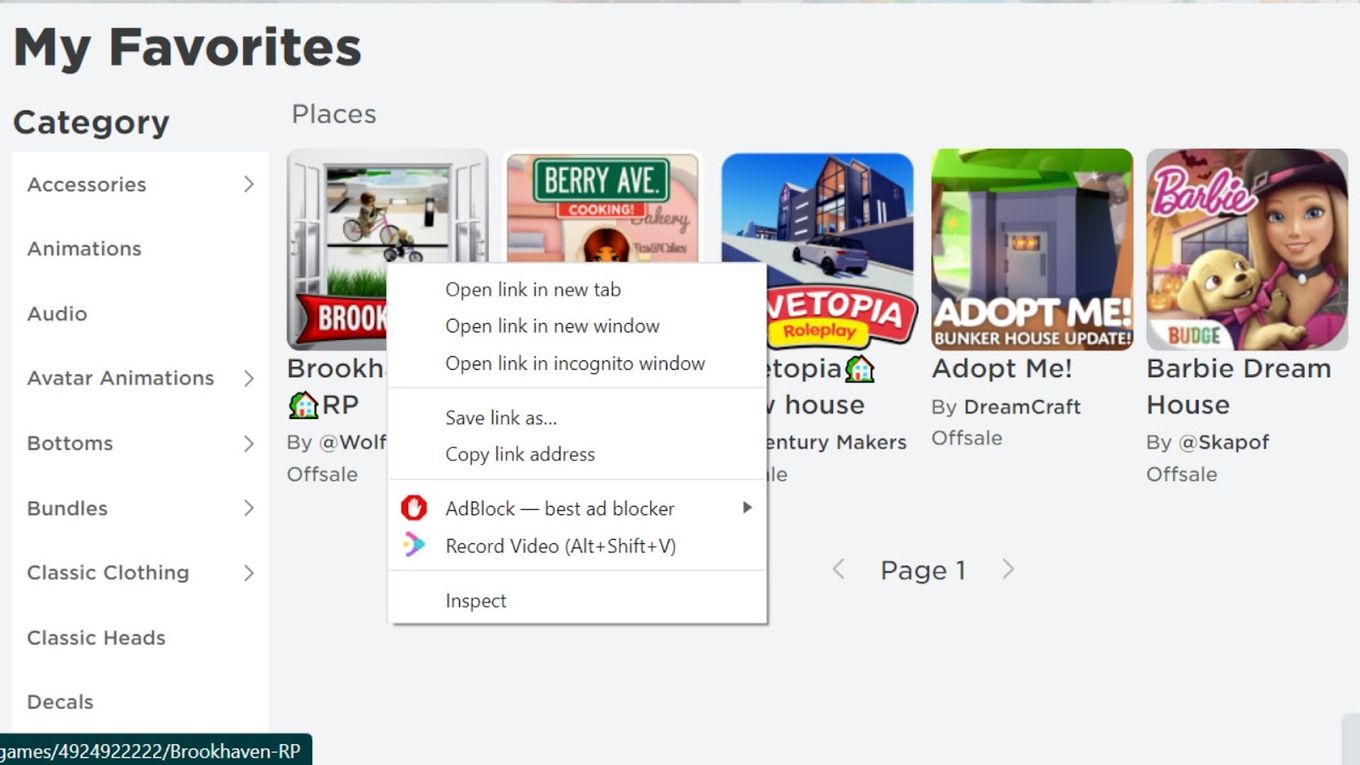A screenshot depicts a visually cluttered webpage showcasing a selection of different games organized under a ‘My Favorites’ header, prominently displayed in large black text at the top left corner. Below this header, a vertical column titled ‘Category’ lists various categories including Accessories, Animations, Audio, Avatar Animations, Bottoms, Bundles, Classic Clothing, Classic Heads, and Decals, all in black text.

To the right of this category list, five game images are arranged in a horizontal row. The first game is titled "Brook..." but the full title is obscured by an open context menu. This context menu offers options such as Open Link in New Tab, Open Link in New Window, Open Link in Incognito Window, Save Link As, Copy Link Address, Add Block, Best Add Blocker, Record Video, and Inspect.

The same context menu partly covers the image of the next game titled “Berry Avenue Cooking,” with only the top part visible. The following game’s title, "VETOPIA Roleplay," is also partially obscured but includes a visible image featuring a house and a car on a road. To the right, the fourth game is titled “Adopt Me: Bunker House Update.” Finally, the last game image features Barbie alongside a puppy, captioned “Barbie Dream House” beneath it.

The interplay of the category list, the partially visible game titles, and the intrusive context menu creates a busily composed screenshot of a favorites page filled with various gaming interests.